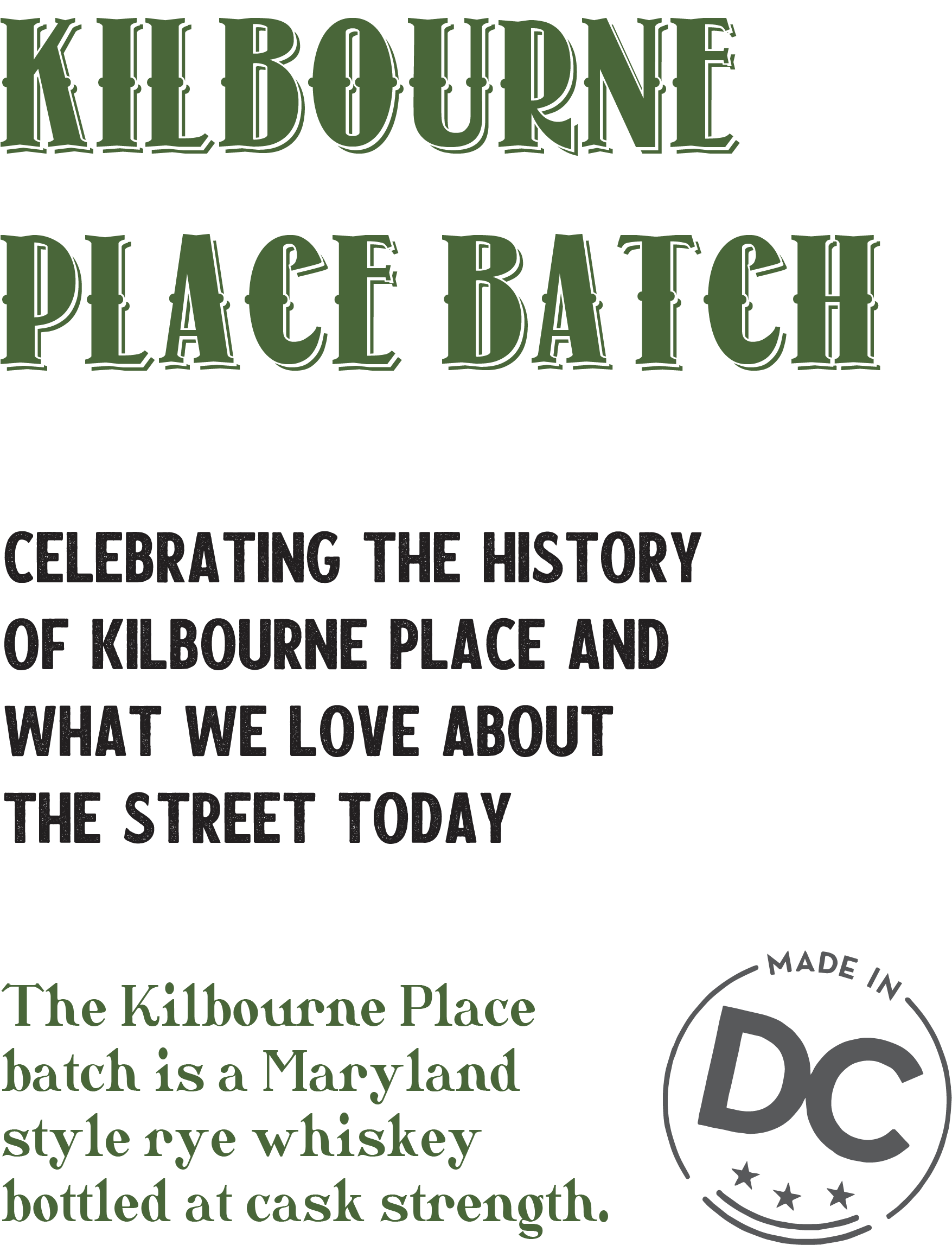This image displays a poster or sign against a white background. At the top, in bold green font with an old-fashioned look, it reads "Kilbourne Place Batch." Below that, in plain black block letters, it states, "Celebrating the History of Kilbourne Place and What We Love About the Street Today." Further down, in a smaller, stylized green font, the text reads, "The Kilbourne Place Batch is a Maryland-style rye whiskey bottled at cask strength." To the right of this paragraph, there's a circular emblem with a lined border, featuring the words "Made In" at the top, "DC" in bold letters in the center, and three stars beneath the "DC."